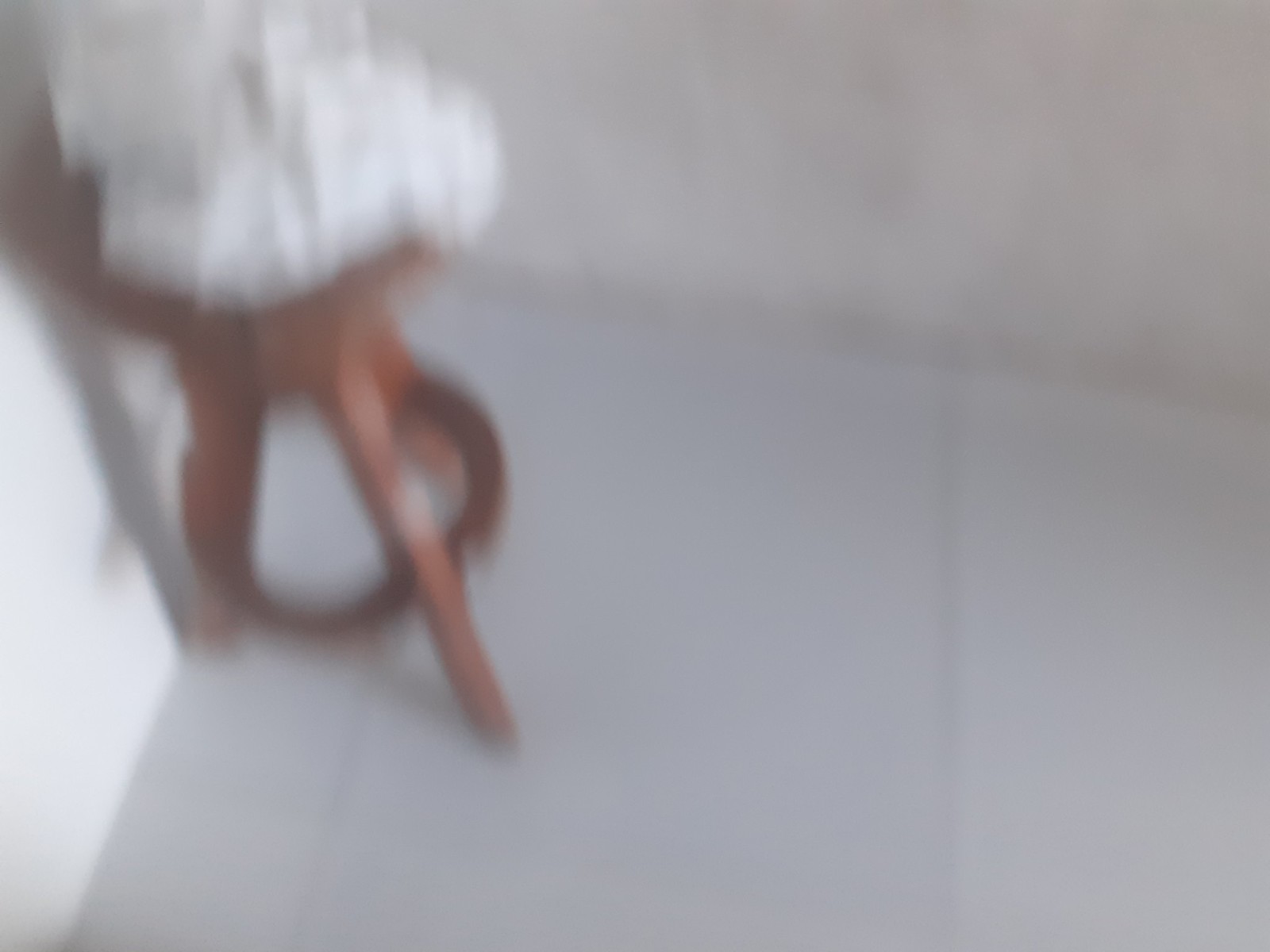In this image, we observe a blurry brown end table positioned in the corner of a room. The table is located on the left-hand side of the frame and features a circular base supported by three diagonally arranged legs. It has a small, circular tabletop upon which rests a light gray and white object, although this object is blurry and difficult to identify. The table casts a subtle shadow to its left.

The room itself is characterized by light gray walls visible along the left-hand side and the upper right portion of the image. The flooring is a light gray, embellished with slight vertical lines that create a patterned effect. This meticulous depiction provides a detailed context of the room's layout and aesthetic features.